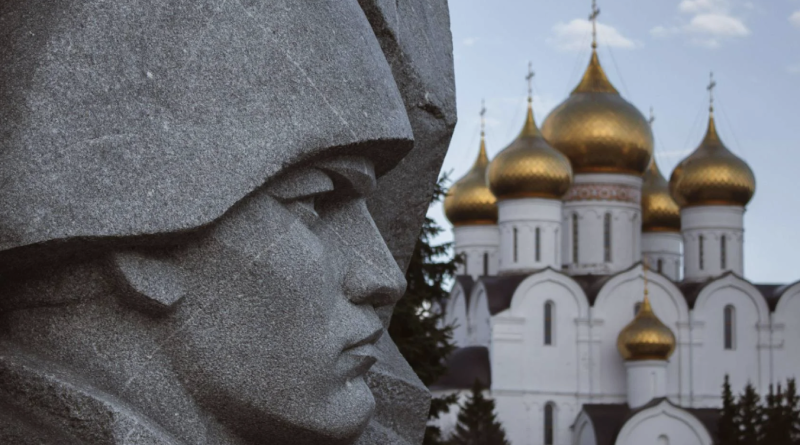This photograph captures a detailed juxtaposition of a stone statue and a grand architectural structure, likely situated in Russia. Dominating the left side of the image, the gray statue represents a stern-faced figure in a military helmet, meticulously carved from weathered stone. Each facial feature—narrowed eye, prominent nose, firmly set mouth, and chiseled chin—exudes intensity, as it faces rightward. The statue appears to be a part of a larger rock formation, blending seamlessly into its rugged surroundings.

On the right side, the composition transitions to an imposing white building, adorned with numerous golden, onion-shaped domes reminiscent of the iconic spires found in Russian architecture. Each gilded dome is topped with a small cross, adding a layer of grandeur to the edifice. The structure, which stretches multiple stories high, features narrow, elongated windows and dark brown rooftops. The building's lower sections are framed by treetops, further enriching the scene with a touch of nature. Above, a light blue sky dotted with drifting clouds provides a serene backdrop to this captivating blend of art and architecture.